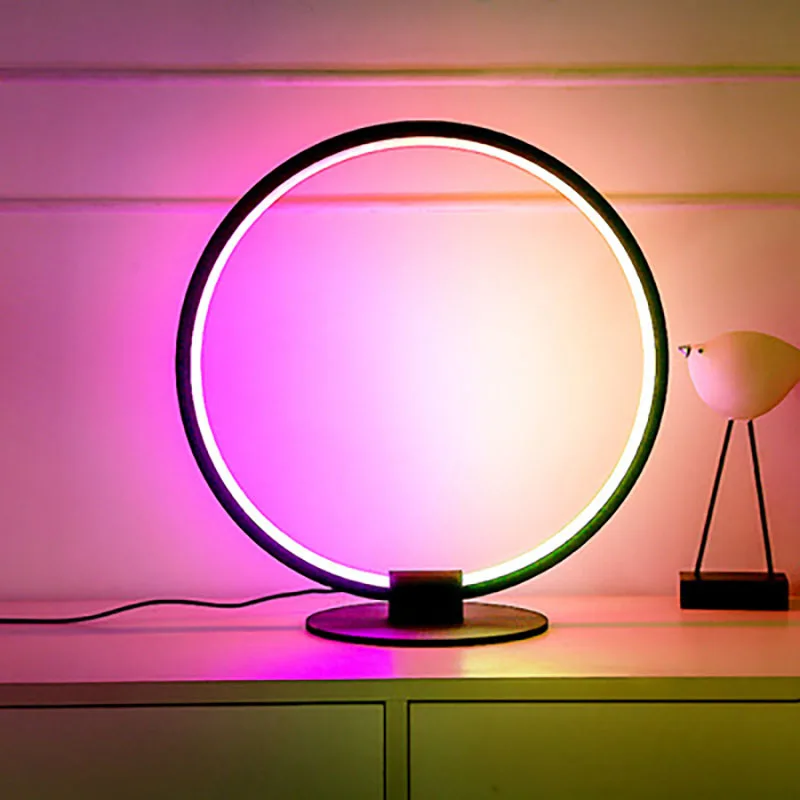The image is set in what appears to be a bedroom, though the exact colors are difficult to discern due to the unique lighting. Central to the composition is a dresser, likely green, though it may appear white or gray in the dim lighting. Atop the dresser sits a large circular ring light, typically used by those in fashion or makeup for optimal facial lighting. This ring light exudes various hues, shifting from pink to purple to orange and white, creating an ambient glow across the room. Adjacent to the ring light is a peculiar bird-shaped knick-knack, which stands on long legs with a black base. The bird features a solid black eye and a detailed beak, contributing to the overall eclectic and moody aesthetic of the scene.